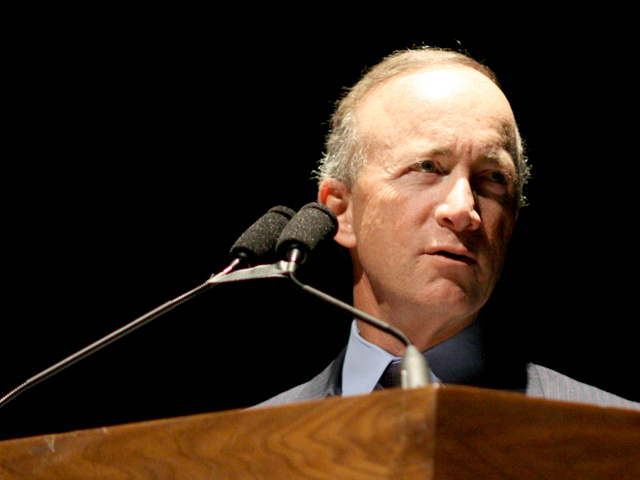This photograph captures Mitch Daniels, an older man with a slender, elongated face, standing behind a brown wooden podium. He is dressed in a darker suit jacket over a light blue dress shirt, complete with a barely visible black tie. His sparsely haired head, slightly balding with gray and blonde thinning hair, is partially illuminated by a spotlight, especially highlighting his large, shiny forehead. Mitch Daniels is looking off to his left, his face divided by a stark shadow on one side and bright light on the other. The podium features two long, black microphones held together at their stems by a band or tape, each topped with larger black pop filters. The backdrop behind him is black, accentuating the dramatic lighting on his face and adding a somber tone to his concerned expression.